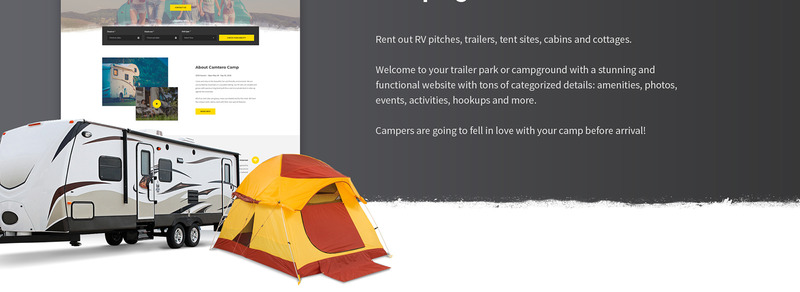The image depicts a modern and expansive website dedicated to the sale of various camping accommodations, including caravans, tents, cabins, cottages, trailers, and pitches. The focal point appears to be a contemporary caravan featuring two doors and a sophisticated palette of white, black, and beige. Ample windows allow natural light to flood the interior, creating a bright and welcoming atmosphere.

Adjacent to the caravan is a vibrant yellow tent, equipped with an overhanging flysheet for weather protection, a zippered entrance, and a small front mat to ensure a clean entry. The image also highlights a trailer with levelling pads at the front for stability. Though the back of the trailer is obscured by the tent, notable features include tandem axles with stylish mag wheels and a set of front lights designed for safe towing.

In the background, there is some small, hard-to-read text, likely containing links to additional sections of the website where users can explore more detailed information about the products offered. This site appears to be a valuable resource for camping enthusiasts, providing a comprehensive selection of gear and accommodations to enhance their outdoor experiences.